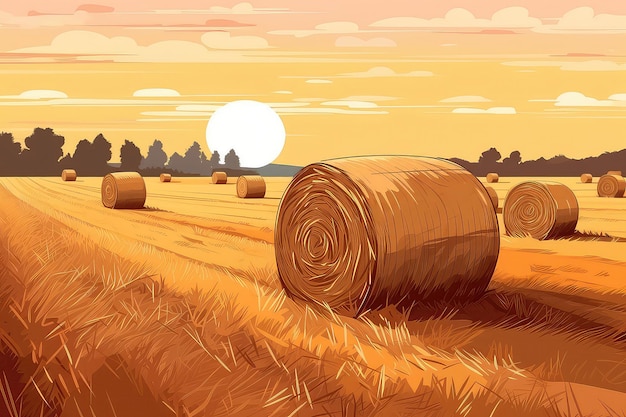The illustration depicts an expansive farm field filled with numerous tightly rolled hay bales. The ground in the foreground is a deep orange, indicative of dry hay or wheat. These hay bales are scattered abundantly across the field. On the horizon, dark brown silhouettes of trees frame the scene, especially prominent on the left and right sides. Centered on the horizon is a large, nearly white sun, suggesting it is either setting or rising. The sky behind the sun transitions from a bright orange near the horizon to pink hues higher up, with horizontal clouds cutting across the canvas. The overall color palette is warm and rich, creating a striking contrast between the dry, golden field and the vivid tones of the sky.